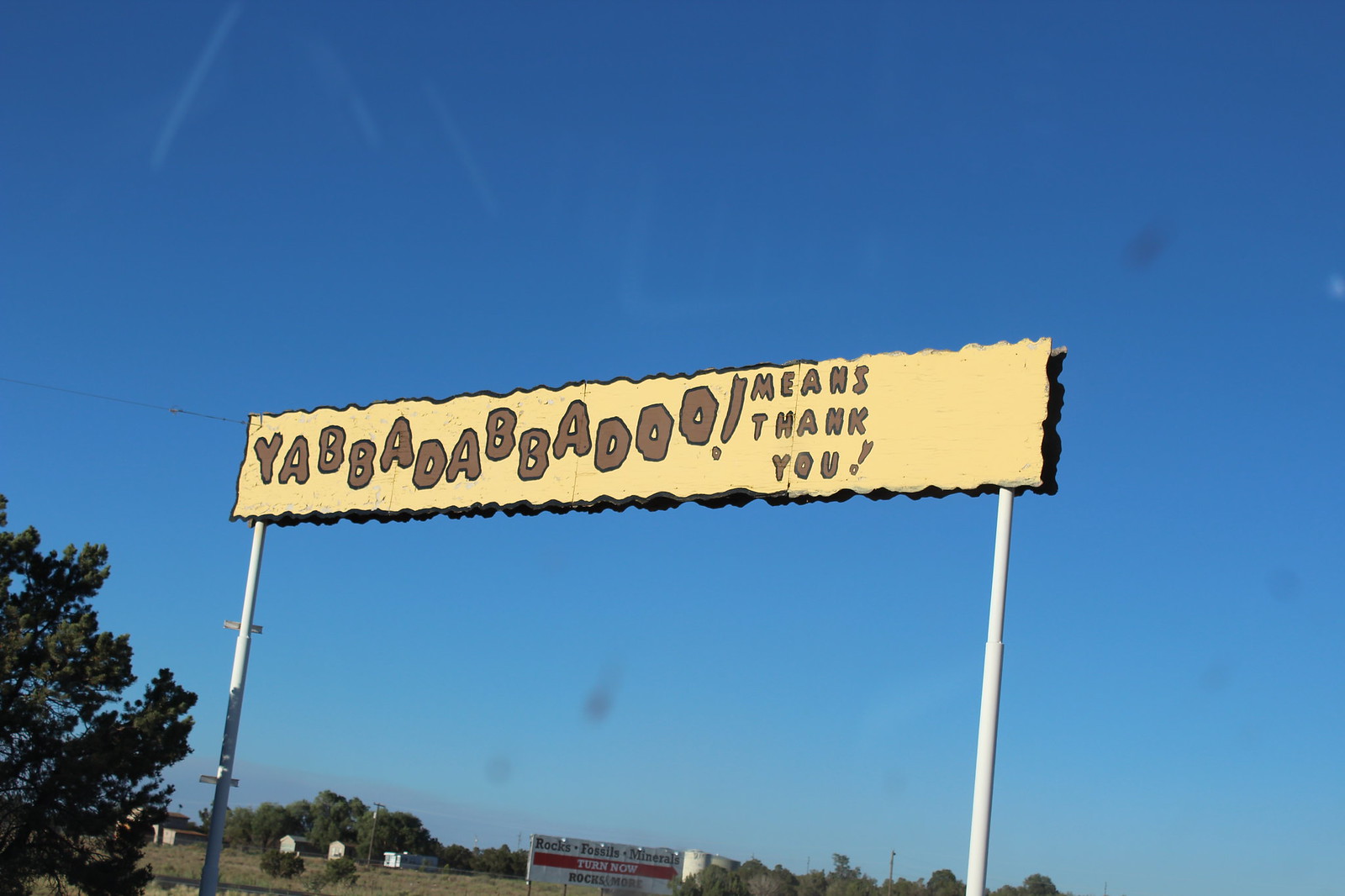This photograph captures a wooden sign mounted on two white poles, taken from the outside of a moving vehicle with some visible dried rain spots on the car window. The sign itself is light yellow and features cartoon-like, dark gray lettering that reads "Yabba Dabba Doo means thank you!" The exuberant exclamation point is prominently placed right after "Yabba Dabba Doo." The right side of the sign remains blank. In the lower left corner of the image, there's a tree partially visible. A portion of another sign, which is white with a red stripe, appears cut off at the bottom center. The background shows open land dotted with more trees, suggesting that this might be a rural or farm setting. The clear sky above showcases a couple of airplane trails, adding depth to the serene outdoor scene.